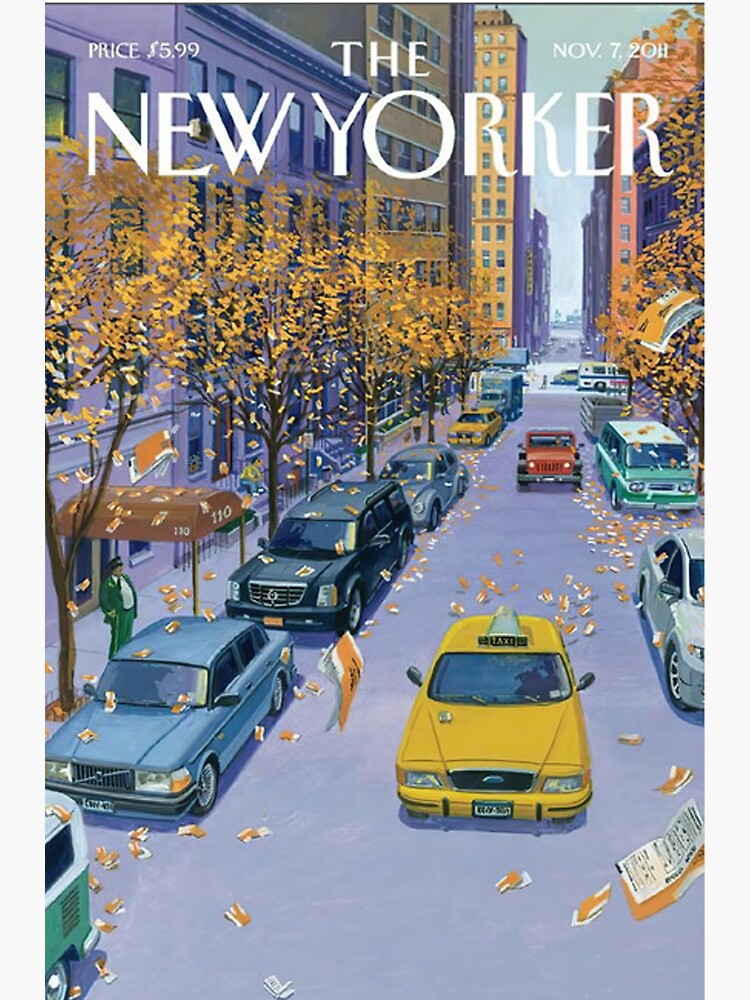The cover of the New Yorker magazine dated November 7, 2011, prominently features a vivid painting of a street scene in Manhattan. The image is bordered by light gray strips on the left and right. Notably, in white print, the magazine's title "The New Yorker" is at the top, with the price "$5.99" in the upper left corner and the date in the upper right. The scene showcases a yellow taxi cab driving toward the viewer in the lower center, followed by a red jeep about 20 feet behind it.

Flanking the street are vehicles parked on both sides beneath narrow-trunked trees shedding their golden leaves, indicating the fall season. Among the parked vehicles on the left are various cars, including a Volkswagen bus and a Lexus. Prominently, a doorman in a green uniform stands beside an orange canopy marked with the building number "110". The canopy is in front of a gray building amid other tall structures that recede into the distant background. The skyline features towering skyscrapers, enhancing the city's urban atmosphere. Alongside the falling leaves, pieces of paper with black print are visible floating in the air, adding a dynamic element to the autumnal setting.